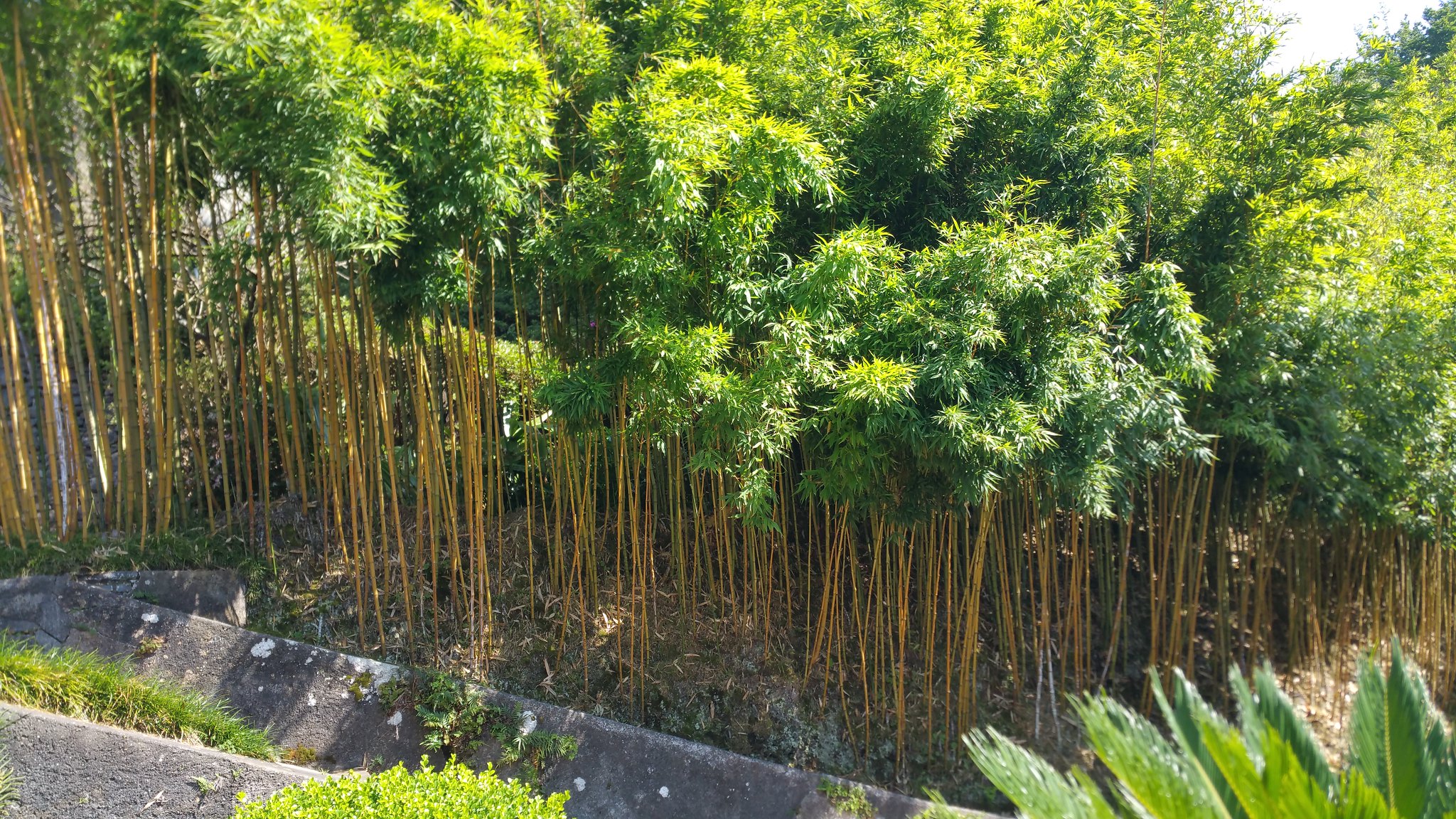The photograph captures a dense grove of tall, bamboo-like plants with thin, yellowish trunks that almost resemble tree branches emerging from the ground. The vibrant green canopy above is lush and sunlit, casting dappled light throughout the grove. In the foreground, two strips of gray concrete are visible, possibly serving as a spillway or walkway, interspersed with patches of dirt and low bushes. The bottom right corner of the image features the edges of green leaves from a nearby plant, providing additional texture and depth to the scene.